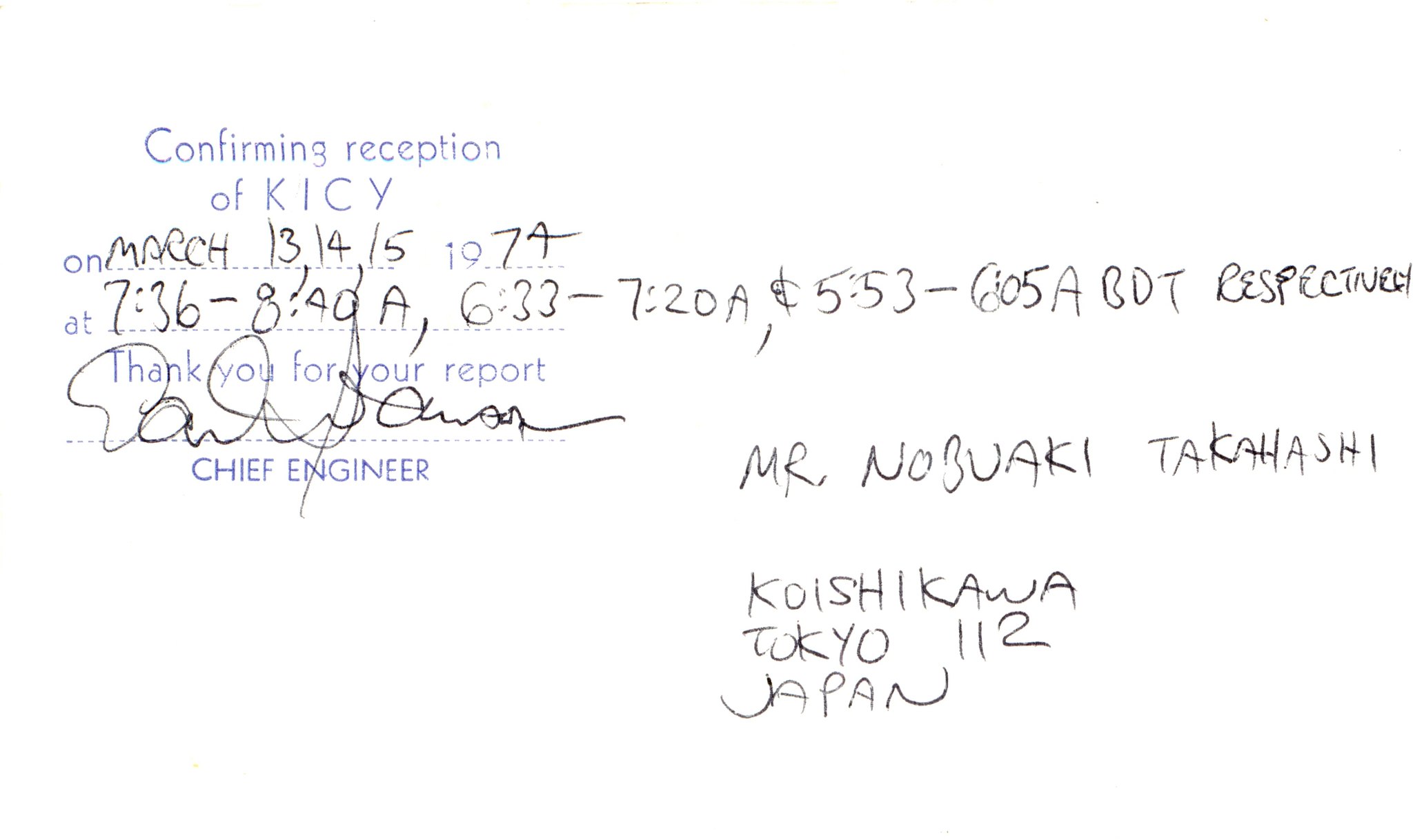The image appears to be a scanned written note or letter confirming the reception of KICY. The text at the top, printed in blue, reads "confirming reception of KICY." Handwritten entries indicate the dates and times of reception: March 13th, 14th, and 15th, 1974, with the times listed as 7:36 to 8:40 A.M., 6:33 to 7:20 A.M., and 5:53 to 6:50 A.M. BDT, respectively. Below this, in printed blue text, it says "Thank you for your report," followed by a signature. "Chief Engineer" is printed underneath the signature. To the right, it is addressed to Mr. Nubaki Takahashi, with his address written as Koshikawa, Tokyo 1112, Japan, in handwritten text. This document appears to serve as a form of acknowledgment or receipt of the information detailed within.